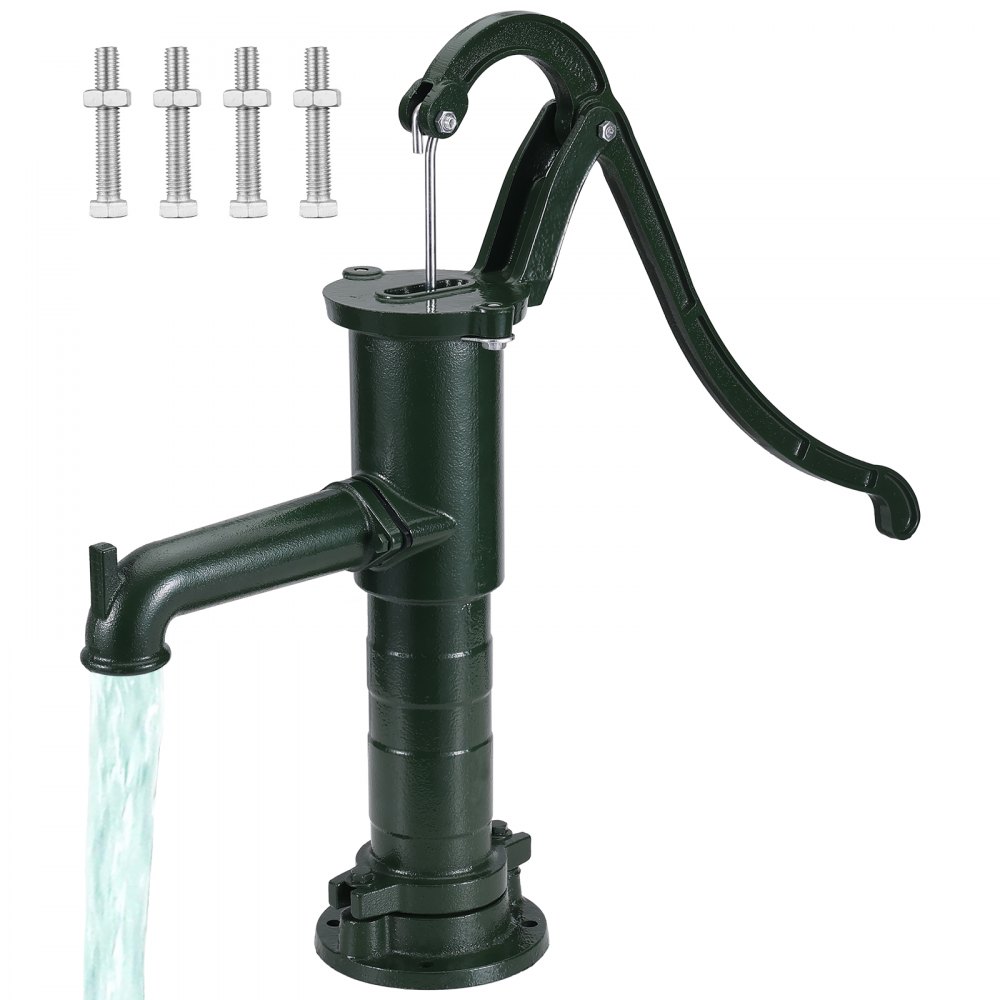This image depicts a glossy black faucet with a design reminiscent of an old-fashioned water pump. The faucet features a long, black metal lever on top, which serves as the pump handle. Attached to the handle is a thin silver hook that extends down into the faucet base. The faucet itself emerges from a vertical black pipe and has a black spout aimed downward, pouring out a steady stream of water. The base of the faucet is equipped with holes that are likely for securing it to the ground or another surface using screws or bolts. In the top left corner of the image, there are four silver nuts and bolts, which may be associated with the installation of the faucet. The background is white, highlighting the intricate details and contrasting colors of the faucet and its components.